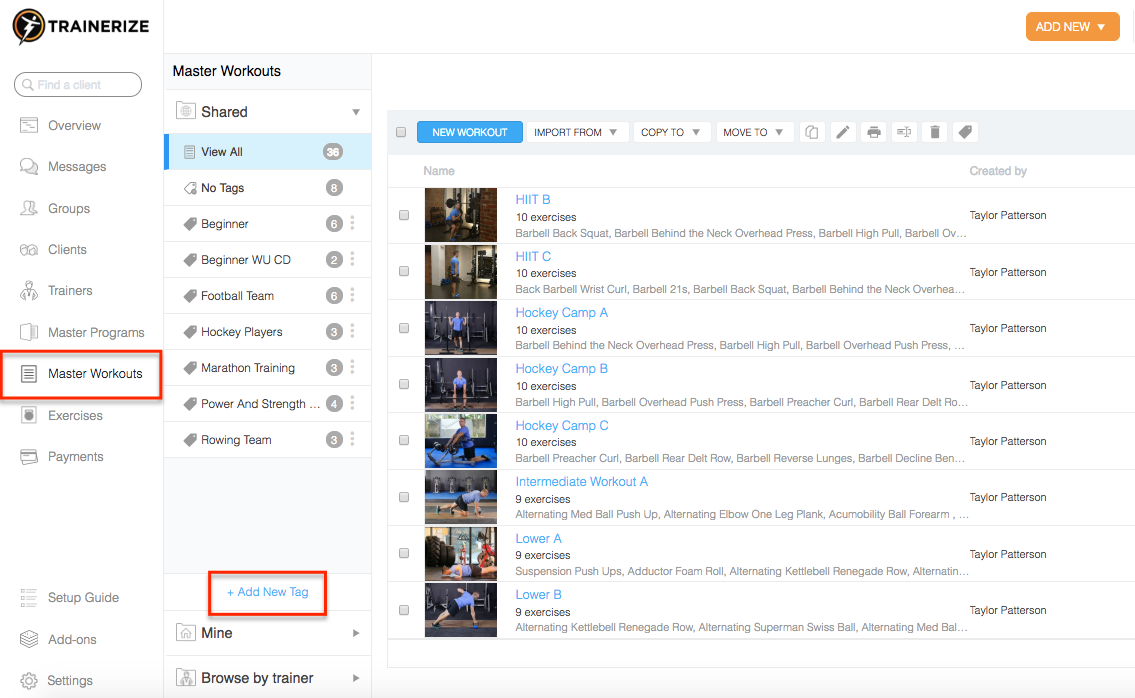Screenshot of the Trainerize workout app interface: 

The image displays the interface of the Trainerize app, recognizable by its logo—a black circle with an inlaid yellow circle near the edge, featuring an icon of a person with wings outstretched and their body shaped like a lightning bolt. 

On the left side, there is a vertical menu with various options: Find a Client, Overview, Messages, Groups, Clients, Trainers, Master Programs, Master Workouts, Exercises, and Payments. At the bottom of this menu, there are additional options for Setup Guide, Add-ons, and Settings. The "Master Workouts" option is highlighted in black and additionally emphasized with a red rectangle around it.

To the right of the menu, under "Master Workouts," several categories are listed: Shared, View All, No Tags, Beginner, Beginner with CD, Football Team, Hockey Players, Marathon Training, Power and Strength, Rowing Team, with an option to Add a New Tag at the bottom in red. The "View All" category is currently selected, displaying a count of 35 workout options. 

Beside this, on the right side of the interface, are various workout options including thumbnails of individuals performing exercises. A blue-highlighted button labeled "New Workout" is present, along with options to Import, Copy, or Move workouts. The thumbnails display a variety of workouts, such as:

- HIIT B
- HIIT C
- HIIT
- Hockey Camp A
- Hockey Camp B
- Hockey Camp C
- Intermediate Workout A
- Lower A
- Lower B

Each workout is created by Taylor Patterson and lists the number of exercises included, with most having 10 exercises and a few having 9. The description for each workout includes the specific exercises, such as Barbell Back Squat, Barbell Behind-the-Neck Overhead Press, Barbell High Pull, Barbell Overhead for the HIIT B workout.